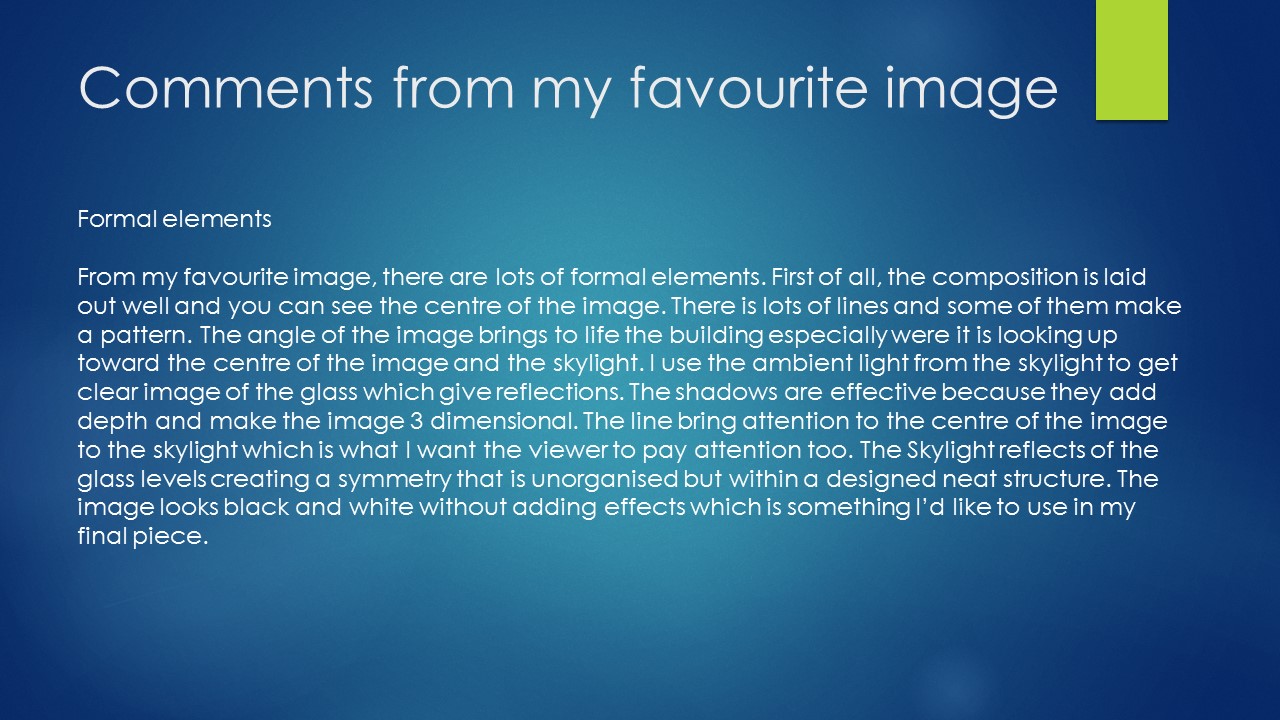The image is a screenshot of a slideshow slide with a blue background and white text titled "Comments from My Favorite Image." In the upper right corner, there is a green rectangle that appears to serve no purpose. The text describes a photograph of a building, highlighting several formal elements. The composition is well laid out, with a focus on the center of the image. Numerous lines create patterns and lead the eye toward a skylight. The angle of the photograph enhances the building's features, using ambient light from the skylight to capture reflections on the glass. Shadows add depth, giving the image a three-dimensional quality. The lines draw attention to the center of the image and the skylight, which reflects off the glass surfaces to create an unorganized yet structured symmetry. The description notes that the image appears almost black and white naturally, an effect the viewer finds appealing for a final piece.